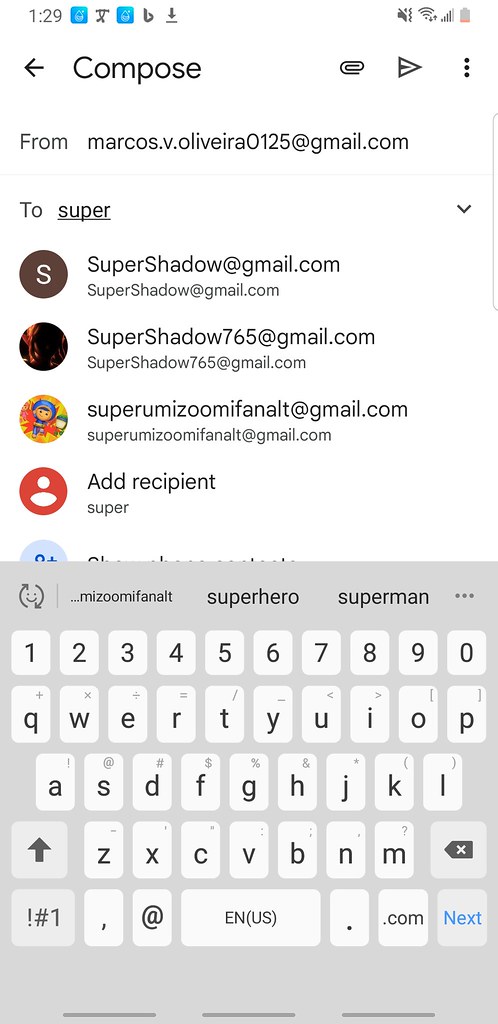The image depicts a vertical phone screen displaying a messaging interface. At the top, the title "Compose" is visible, indicating that the user is in the process of drafting a new message. The sender's email address, "marcos.v.olivera0125@gmail.com," is visible in the "From" field. The recipient field is designated as "To: super," which is underlined.

Below the recipient field, there are four suggested contacts listed, all beginning with "super":
1. supershadow@gmail.com
2. supershadow765@gmail.com
3. superamizumfanalt@gmail.com

A prominent red button labeled "Add Recipient" is situated beneath the list of contacts. Further down the screen, the keyboard is displayed, suggesting that the user is in the midst of composing their message. The specific recipient remains unclear due to all contacts beginning with "super."